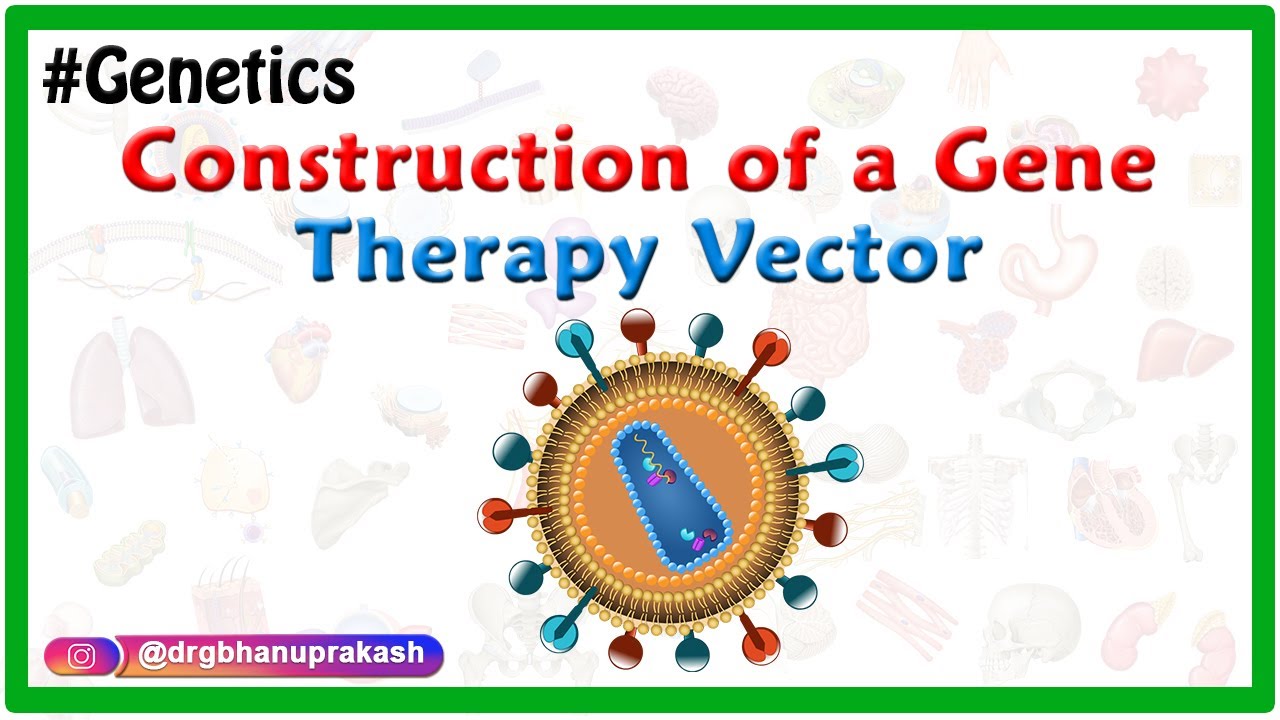This image is a detailed advertisement poster with a green border. The top left features the hashtag "#genetics" in black font. Centered prominently are the phrases "construction of a gene" in red embossed letters and "therapy vector" in blue embossed letters. The main visual element is a circular, yellowish center representing a gene, from which various colored stems—amber, green, blue, red, and each with marble-like ends—protrude, resembling bobby pins. The background subtly displays faded shapes reminiscent of body organs. In the bottom left corner, there's an Instagram advertisement featuring the Instagram logo and the handle "@drgbhanuprakash" in white font.